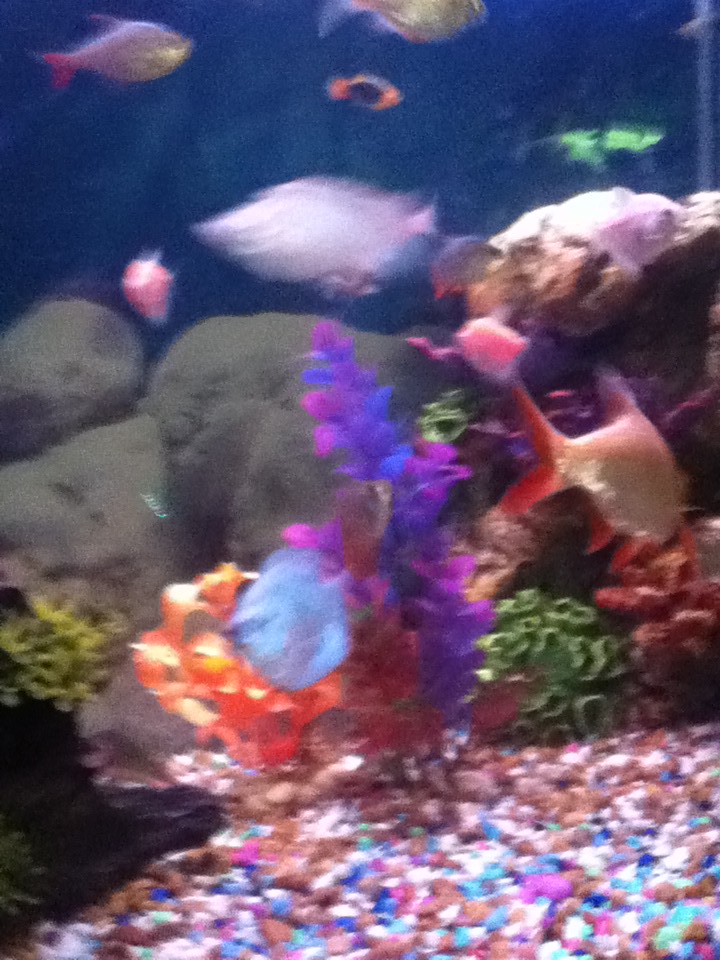An underwater photograph with a solid dark blue background, capturing a colorful and bustling aquarium. This portrait-oriented, albeit blurry, image features a variety of vividly colored fish, including an orange and black fish, a light pink fish with red tips, a bluish one with a red tail, and silvery neon tetras with red tails. At the bottom resides a detailed and colorful array of pebbles in hues of white, blue, pink, and orange. Among the pebbles, there are distinct large gray rocks—one smooth and the other textured—and an assemblage of artificial coral in green and red. Additionally, there’s a vibrant pink-purple-red plant emerging from the rocks and some green algae adding a natural touch. On the left side, a large gray formation resembling oversized mushrooms or bushes provides an imaginative focal point, enhancing the aquatic scene’s complexity and intrigue.